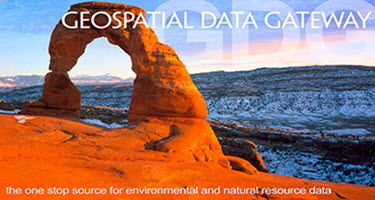The advertisement features a captivating photograph taken from a rocky hill composed of red clay, showcasing a striking natural stone arch that frames the scene. The hill abruptly drops off into a cliff, revealing a breathtaking valley blanketed in snow. The snow extends to the mountains in the distance, which also harbor patches of green trees. Overlaid in white letters across the top of the image, the text reads "Geospatial Data Gateway." At the bottom, in smaller white letters, the caption states, "The one-stop resource for environmental and natural resource data." The overall scene and text highlight the integration of natural beauty and the promise of accessible, comprehensive data in one view.